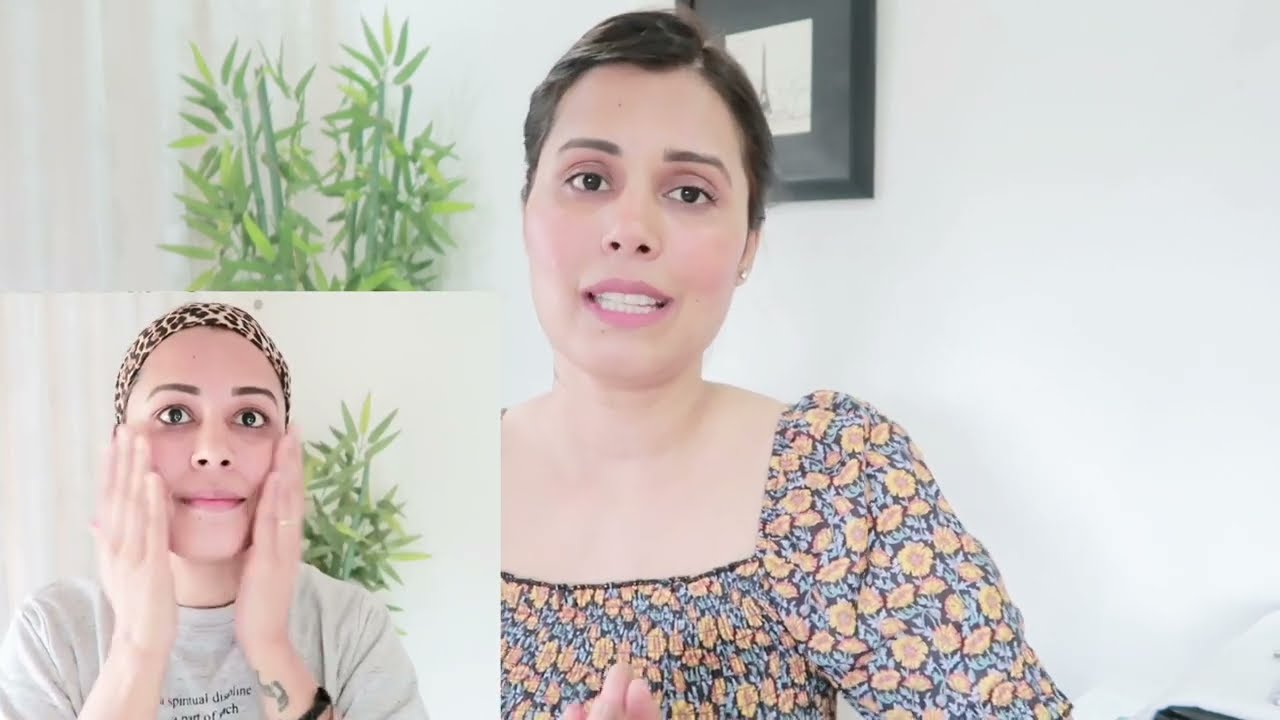The image features a centrally positioned pale-skinned woman with short, neatly parted brown hair and well-groomed eyebrows. She wears subtle pink lipstick and blush that give her a neutral but still distinctly feminine appearance. In the larger, central part of the photo, the woman is smiling with her teeth visible and is wearing a scoop-neck top adorned with vibrant orange flowers and scattered blue leaves. The setting appears to be indoors, likely during the day, with various objects in the background, including a plant and a picture.

In the bottom left corner, there's a smaller inset image of the same woman, now wearing a leopard print hairband and a gray t-shirt. In this inset, she is seen patting her face with both hands, seemingly applying face cream or makeup, and smiling softly without showing her teeth. Surrounding the woman are additional colors like white, brown, tan, gray, green, blue, orange, pink, black, and white, accentuating the details and depth of the photo.